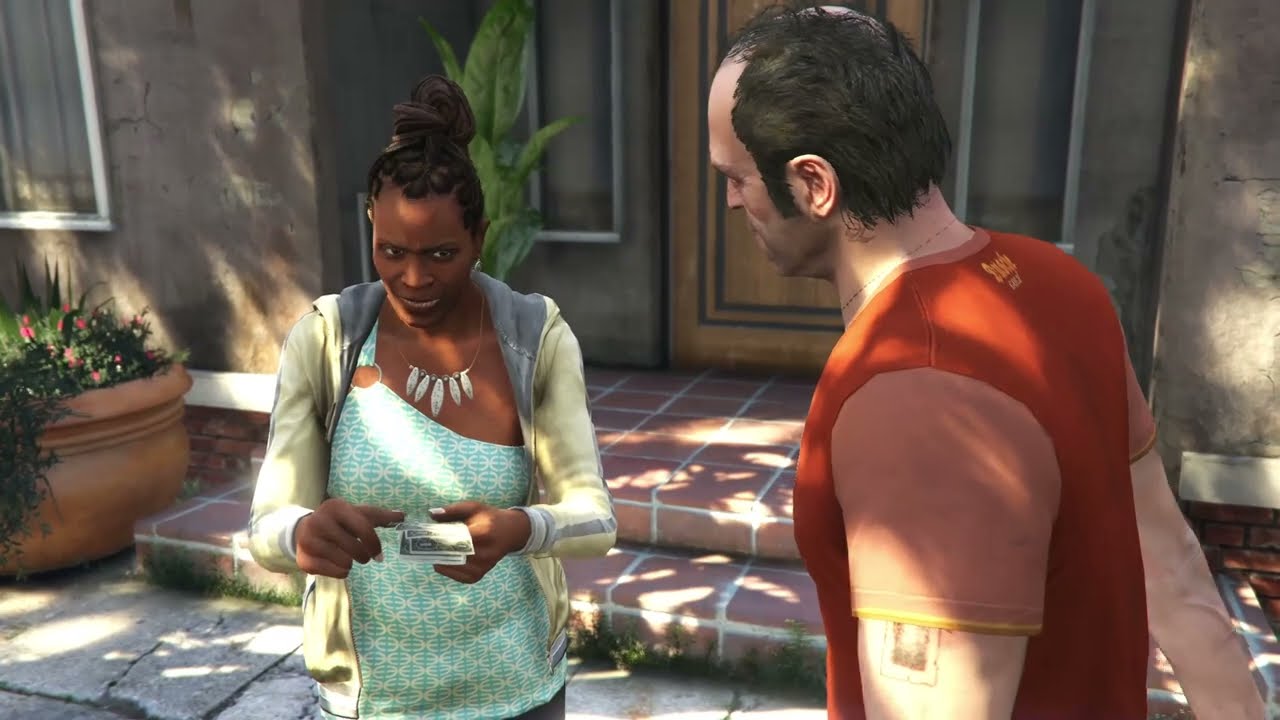In this highly detailed screenshot from Grand Theft Auto V, the animated characters are set on the front porch of a building with a brick staircase, its walls a general shade of gray. On the right stands Trevor, a Caucasian male distinguished by his receding dark brown hair, bald spot at the crown, and sideburns. Trevor sports an orange shirt with salmon-colored sleeves and has a barbed wire tattoo around his neck, partially visible underneath. Facing him is a black female character with dreadlocks tied into a bun atop her head. She wears a single-strapped teal shirt adorned with a shell necklace, further layered with a yellow hoodie featuring a gray interior. The woman, holding a stack of cash about an inch thick, glances at Trevor with a somewhat sheepish expression, making eye contact only from the corners of her eyes. Her demeanor hints at a mix of hesitation and discomfort during their interaction.